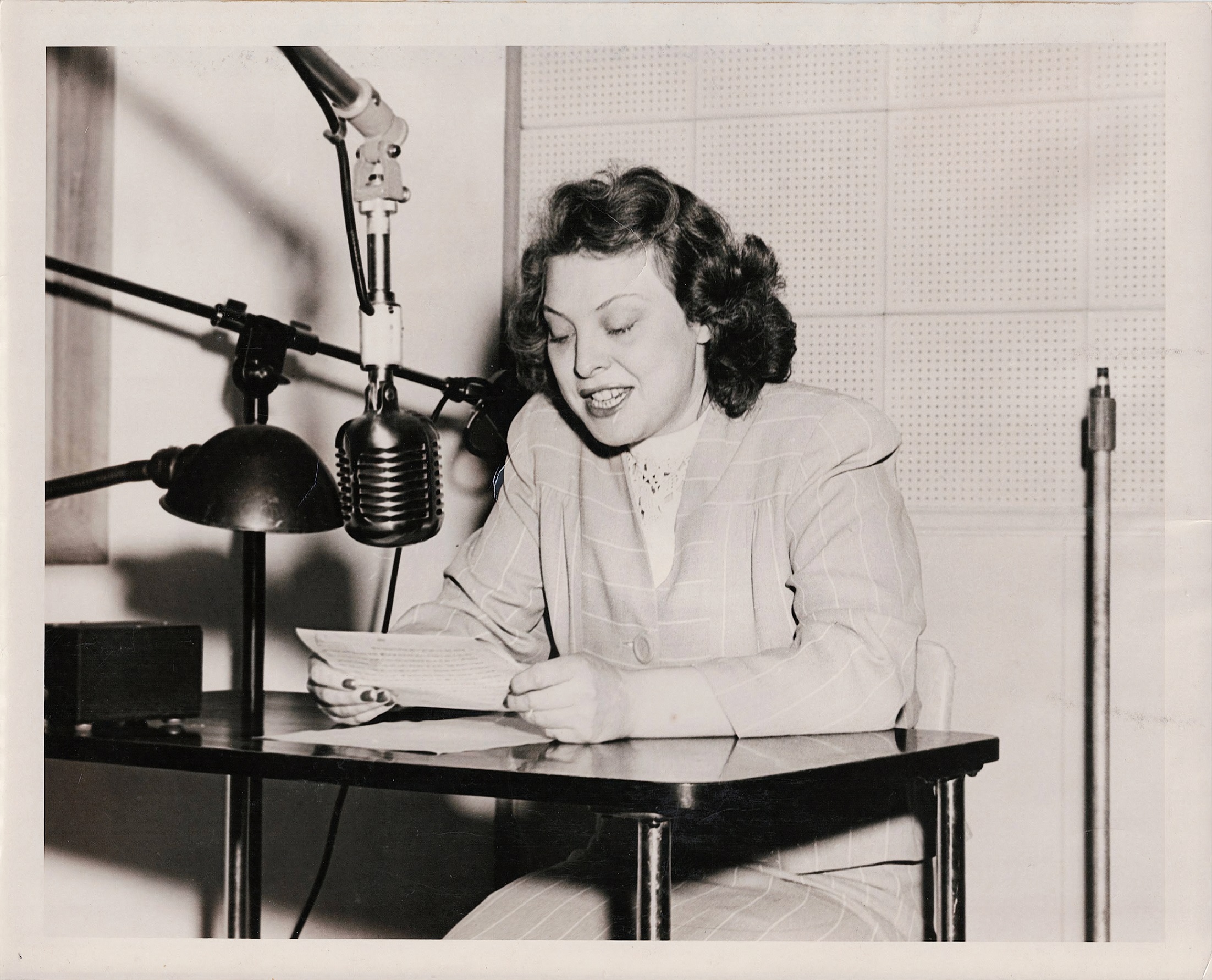In this vintage black and white photo, a woman with short, dark brown curly hair is seated at a smooth black desk, appearing to be a radio broadcaster. She is positioned in front of a microphone mounted on a tripod stand, with a pegboard wall serving as the backdrop. The woman, possibly reading a script as she speaks, is dressed in a professional attire featuring a plaid suit jacket with lines, shoulder pads, and a white shirt underneath. She is also wearing a matching skirt. Her lips and nails are painted a striking red, adding a hint of color to the monochrome image. On the desk, in addition to the script she’s holding, there is another sheet of paper and a box, possibly a radio. An additional microphone stand and a lamp are also visible in the scene.